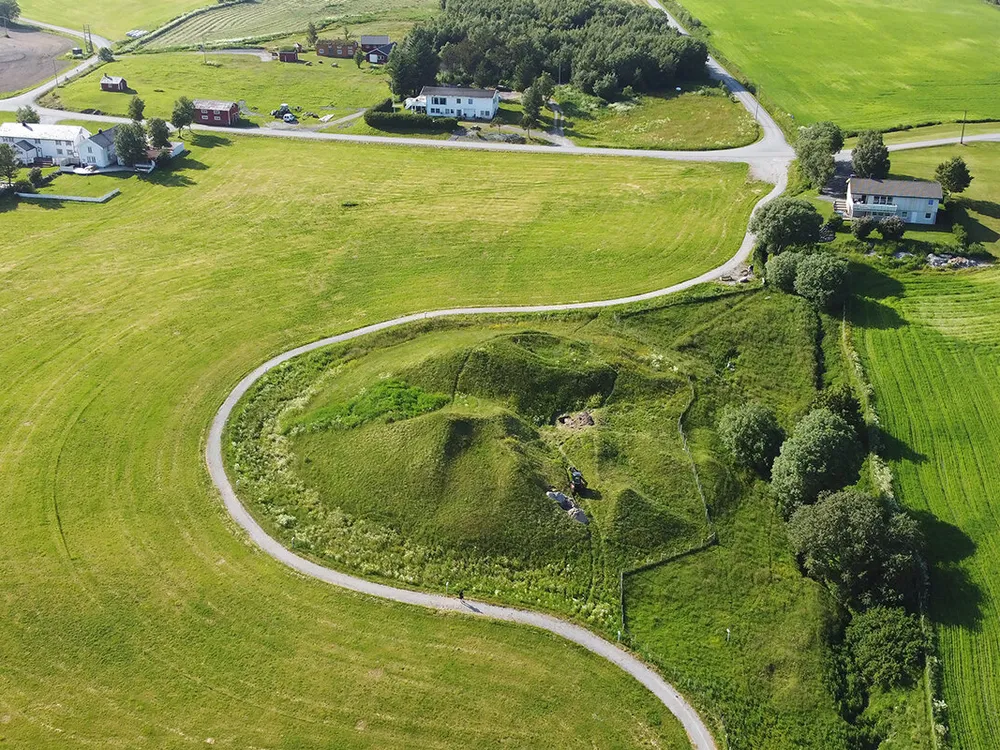An aerial photograph captures a sprawling rural landscape, dominated by lush green fields and interspersed with clusters of large, white and brown rectangular houses. The centerpiece of the image is a large, man-made hill or mound, noticeably indented at the center, possibly remnants of ancient ruins. Encircling the mound is a protective fence, with an asphalt road looping around it, creating a central hub that stretches into three directions. One route leads off-screen to the right, another extends past a dense copse of trees to the top, and the third veers left, passing by more houses. The fields and meadows, dotted with people and cars navigating the roads, reflect a picturesque, sunny day, showcasing both natural beauty and the structured layout of this scenic, rural area.